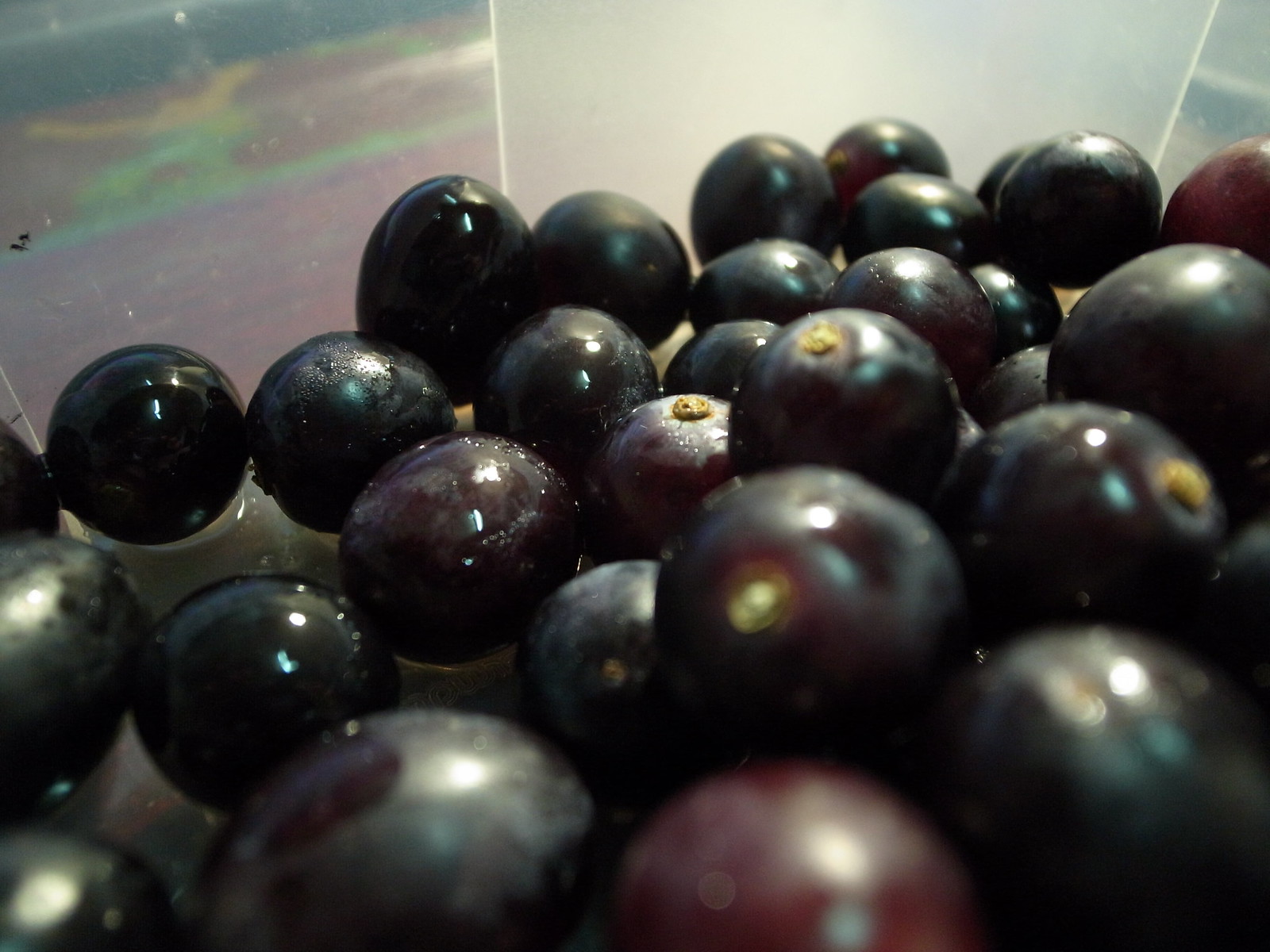This is a close-up image of a dark-colored, round fruit that appear to be either blackberries or purple grapes, housed in a translucent, possibly octagonal-shaped plastic container. The fruits are submerged in a small amount of liquid, likely indicating they have been freshly washed. Most of the fruits are a deep, dark hue, while some exhibit a reddish tint. Each fruit features a small stem at one end. There's a notable opaque reflection visible on the upper left side of the container. The overall appearance suggests the fruit is fresh and well-ripened.